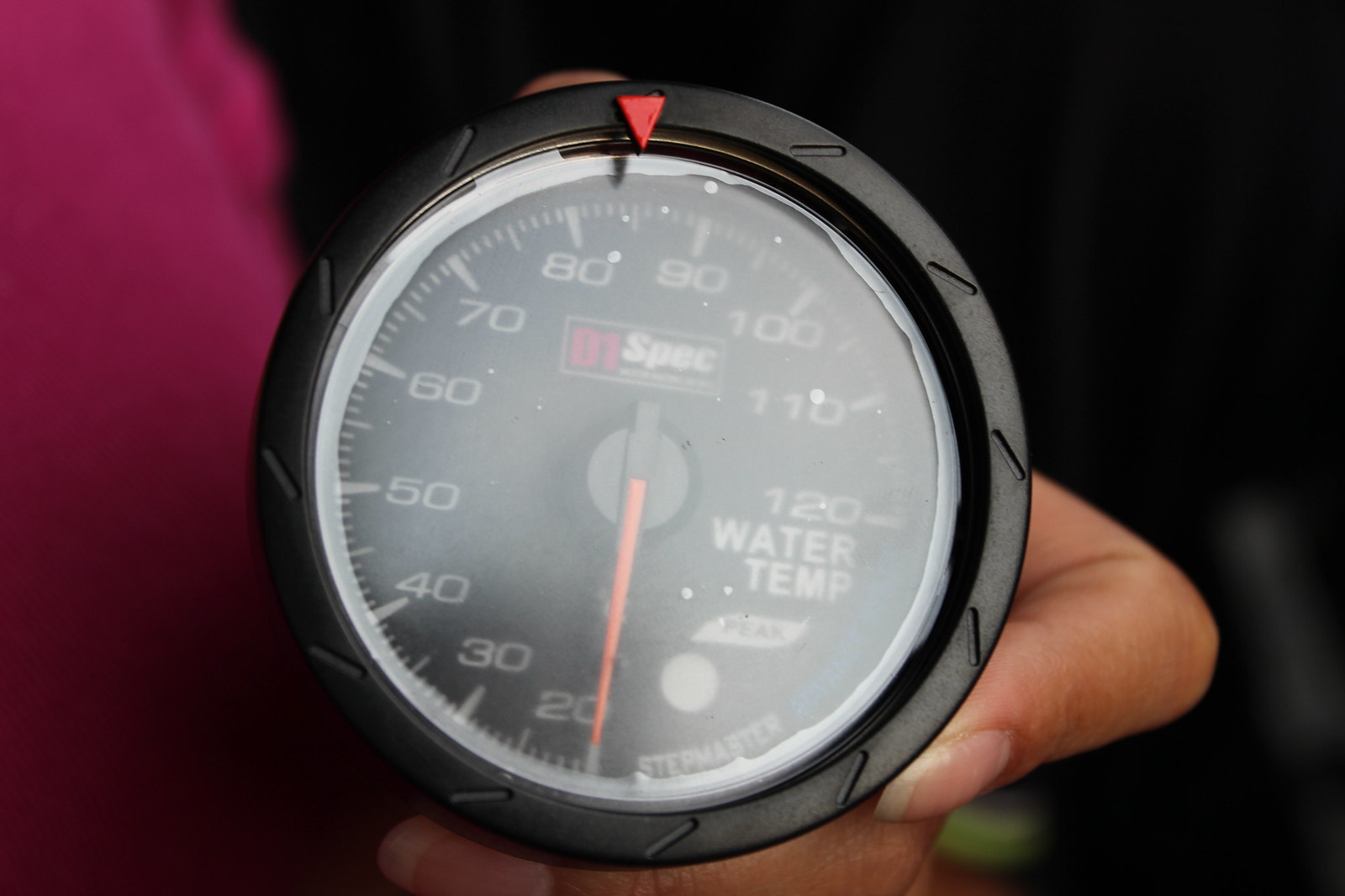In this detailed photograph, a lady with brown skin is holding a device that measures water temperature, often mistaken for a stopwatch. Her long fingernails, predominantly visible on her index and middle fingers, curve around the black instrument. The device features a red, upside-down triangle pointer and an orange needle indicating the water temperature, which presently reads zero, suggesting it is not in use. The lower right section of the device displays the words "water temp" in white text. Additionally, the top middle part of the device shows a partially obscured logo that reads "O1" in red and "spec" in white, though further details are obscured by glare. The lady is partially visible on the left side of the frame, adorned in a sizable jacket in shades of pink or violet. The background remains largely indistinct and black, drawing focused attention to her hand and the water temperature device.